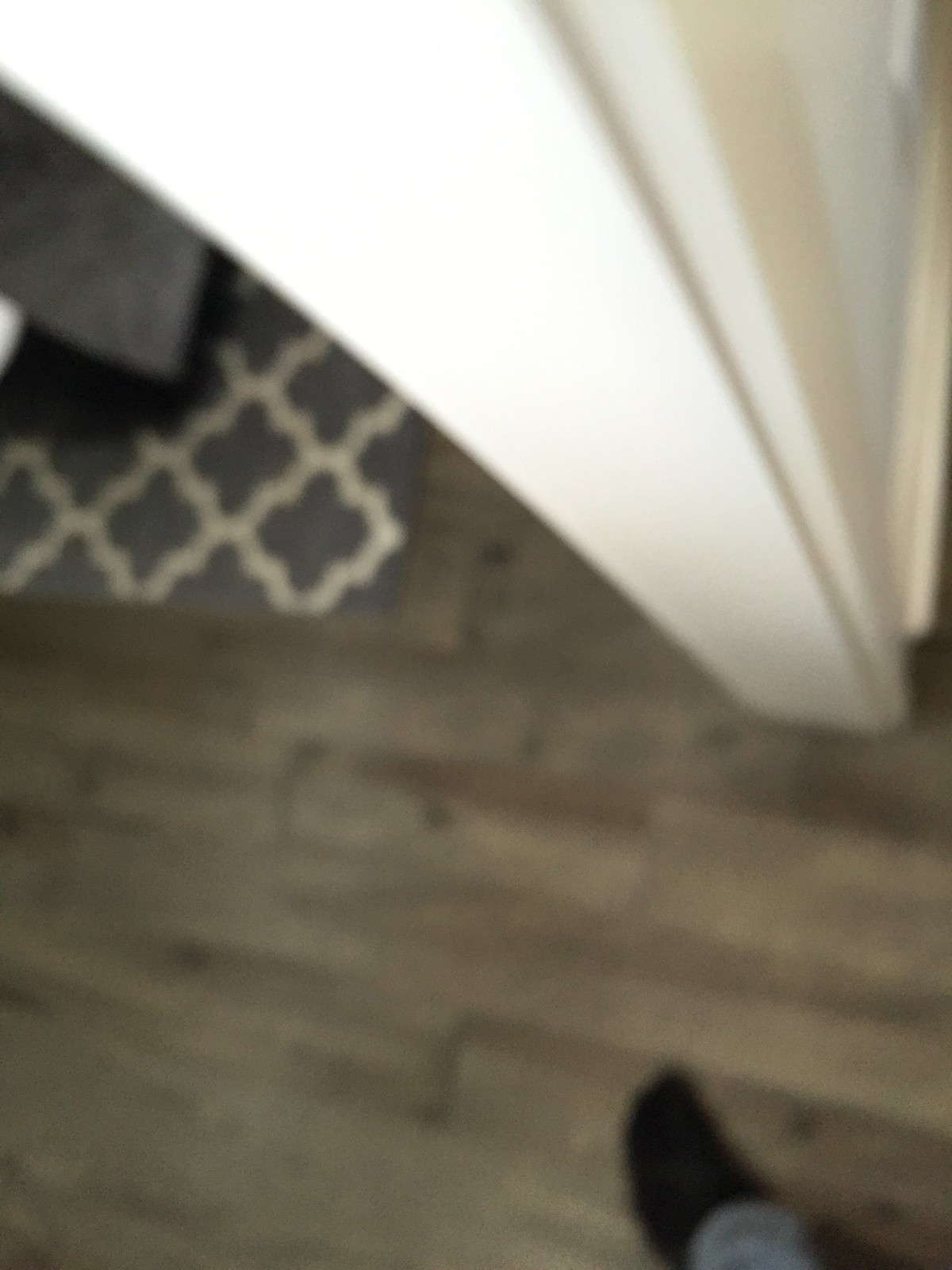The image is a vertically-oriented, blurry photo capturing the lower portion of what appears to be an interior space. The floor consists of dark wood panels arranged horizontally, though the right side is slightly tilted downward, creating a mild inconsistency in alignment. In the upper left corner, a dark blue rug adorned with a wavy diamond pattern is partially visible, overlaying the wooden floor. The lower right corner features a foot clad in a black shoe, with light gray pants extending toward the shoe. Additionally, an off-white door casing is present in the foreground, suggesting the viewer is in the process of transitioning between rooms. The blurred nature of the image implies motion, as even stationary objects appear unclear.